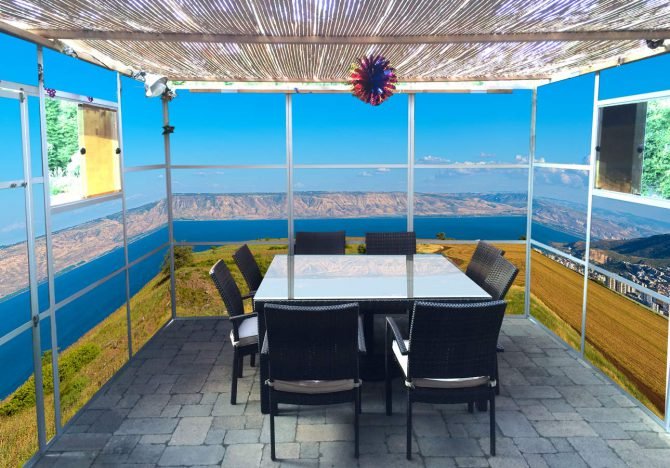The painting captures an immersive sunroom or deck entirely enclosed by glass, supported by a grid of metallic posts. Central to the scene is a square table with a pristine white tabletop, encircled by eight sleek black chairs, which evoke an office-like aesthetic. The table stands on a mosaic stone floor, contributing to the room's minimalist yet modern vibe. The sunroom is bathed in abundant light, highlighting a vast and vibrant landscape visible through the transparent walls. 

In the distance, a large body of water, possibly a lake or ocean inlet, stretches towards mountainous terrain, all under a brilliantly blue sky dotted with a few wispy white clouds. The right side of the image hints at buildings or a town below, while the left side features pictures adding a decorative touch to the glass enclosure. The ceiling is thatched, with horizontal lines tracing across the room, and a colorful hanging item adds a touch of whimsy above the table. The panoramic view outside includes pinkish hills and valleys, enhancing the serene and expansive feeling of the scene. This detailed depiction underscores the blend of indoor comfort with the beauty of the natural world viewed through the encasing glass.